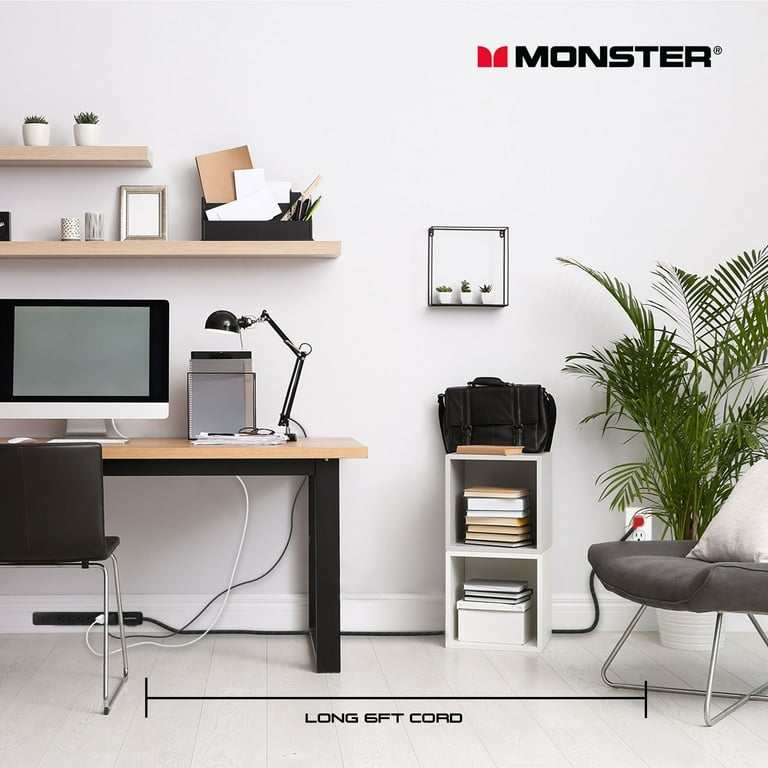This image is an advertisement for Monster Cables, depicting a meticulously arranged office space. Central to the room is a wooden desk with black legs, supporting a computer monitor, a black study lamp, stationery items, and scattered papers. In front of the desk is a small black computer chair. To the right, there's a second chair with a grey seat cushion, a white back cushion, and silver legs, positioned near a prominent indoor plant in a white pot. The floor is grey, contrasting with the white walls that feature various wooden shelves adorned with small plant pots, a mirror, a black box with stationery items, and other decorative artifacts.

A black cord, described in the advertisement as a "long six-foot cord," stretches from an outlet beneath the desk to the chair on the right side, marked by a black line and text indicating its length. The advertisement prominently displays the Monster logo, with its red emblem, in the top right corner. Further, a surge protector and an outlet with a red male connector are visible at the base of the wall, reinforcing the functionality and reach of the Monster cable being advertised. This setup illustrates how the cable can efficiently connect devices over considerable distances, enhancing office organization and convenience.